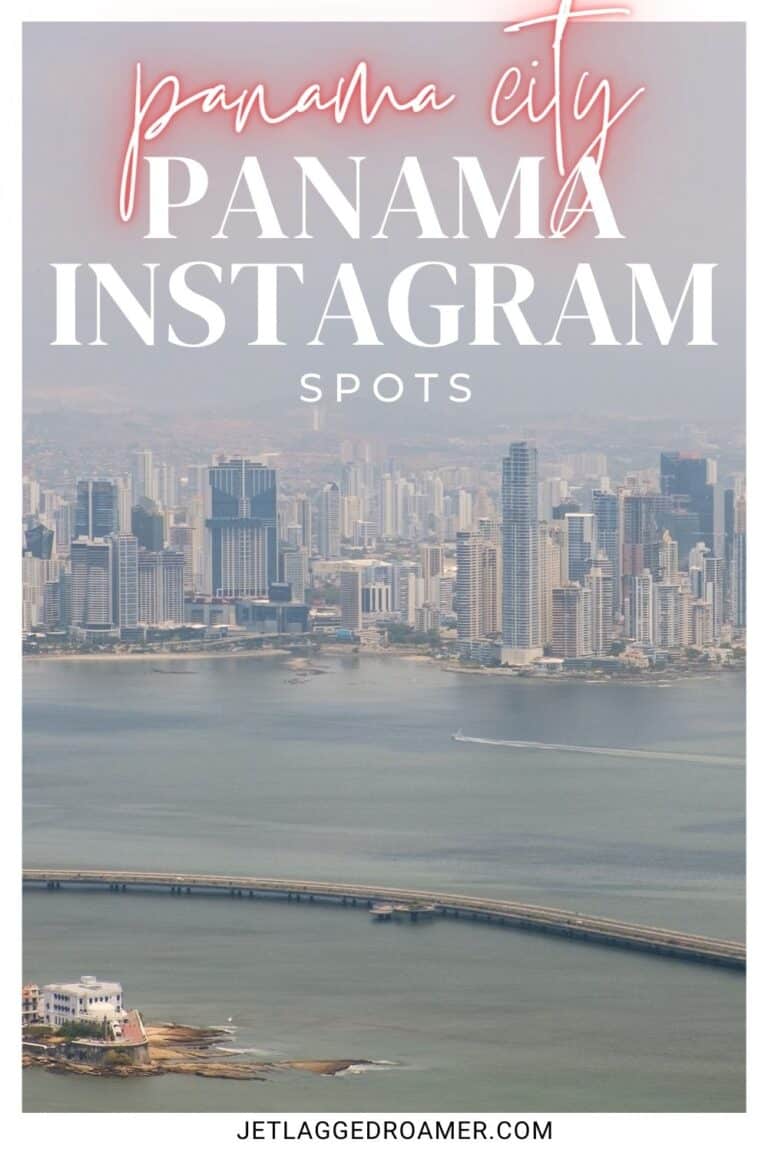The image features the text "Panama City" prominently at the top, rendered in a neon-like cursive font in white with a reddish glow around the letters. The "T" in "City" is particularly exaggerated, extending beyond the top edge of the image. Encasing the entire image is a white border.

Just below this title, in bold, uppercase white text, is the phrase "PANAMA INSTAGRAM." In slightly smaller text beneath that, it reads "SPOTS."

The lower half of the image showcases a stunning cityscape of Panama City in portrait orientation, featuring a skyline filled with numerous towering skyscrapers. The view includes a scenic bay area with an ocean visible and a boat leaving a trail behind it. A long road stretches across the water, and an island with a white building can be seen, with the brown dirt of the island providing a contrasting backdrop.

At the very bottom of the image, "jetlaggedrumor.com" is written in black text.